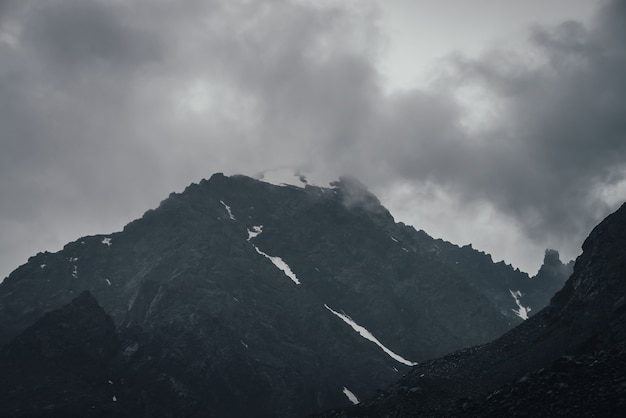In this black and white photograph, a dramatic mountainous landscape is showcased under grim weather conditions. Dominating the center background is a towering, dark, rocky mountain, its peak shrouded in thick, stormy clouds. The upper slopes of the mountain, although partially hidden by mist and clouds, display patches of snow cascading diagonally down one side, suggesting recent snowfall. The sky ranges from white to various shades of gray, with darker clouds clustering ominously near the mountain's pinnacle. In the foreground, a smaller mountain or rocky formation appears, sharing the dark, ashy texture reminiscent of pumice stone, giving the scene a volcanic ambiance. The valley between these two mountains is clearly visible, where the somber atmosphere intensifies the rugged beauty of the terrain. The overall scene feels on the verge of a storm, enhancing the moodiness of this captivating, grayscale image.